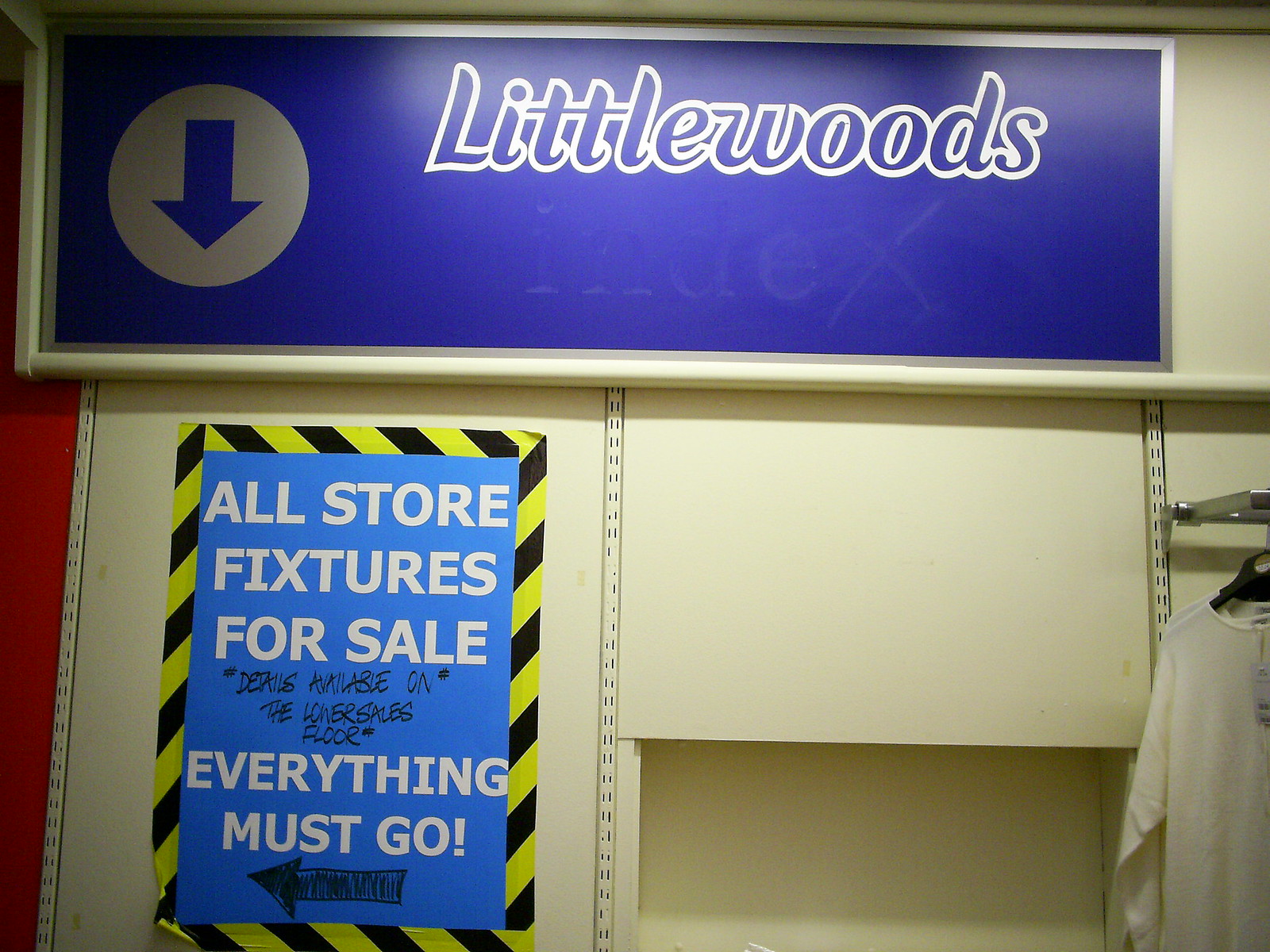In the photograph taken inside a store, the close-up captures the off-white wall at the back adorned with metal fixtures potentially for shelves. Dominating the scene is a large blue sign outlined in silver, featuring a white circle with a blue downward-pointing arrow. Beside this symbol, the stylized, blue-with-white-outline text reads "Little Woods." Below this sign, a prominent blue banner bordered with yellow and black diagonal caution stripes displays urgent white-and-black text, stating "All store fixtures for sale. Everything must go." Additionally, there is handwritten information in black marker mentioning details available on a specified floor, accompanied by a black arrow pointing left. On the right edge of the image, a metal rack is partially visible, holding a black hanger with a white t-shirt draped over it.